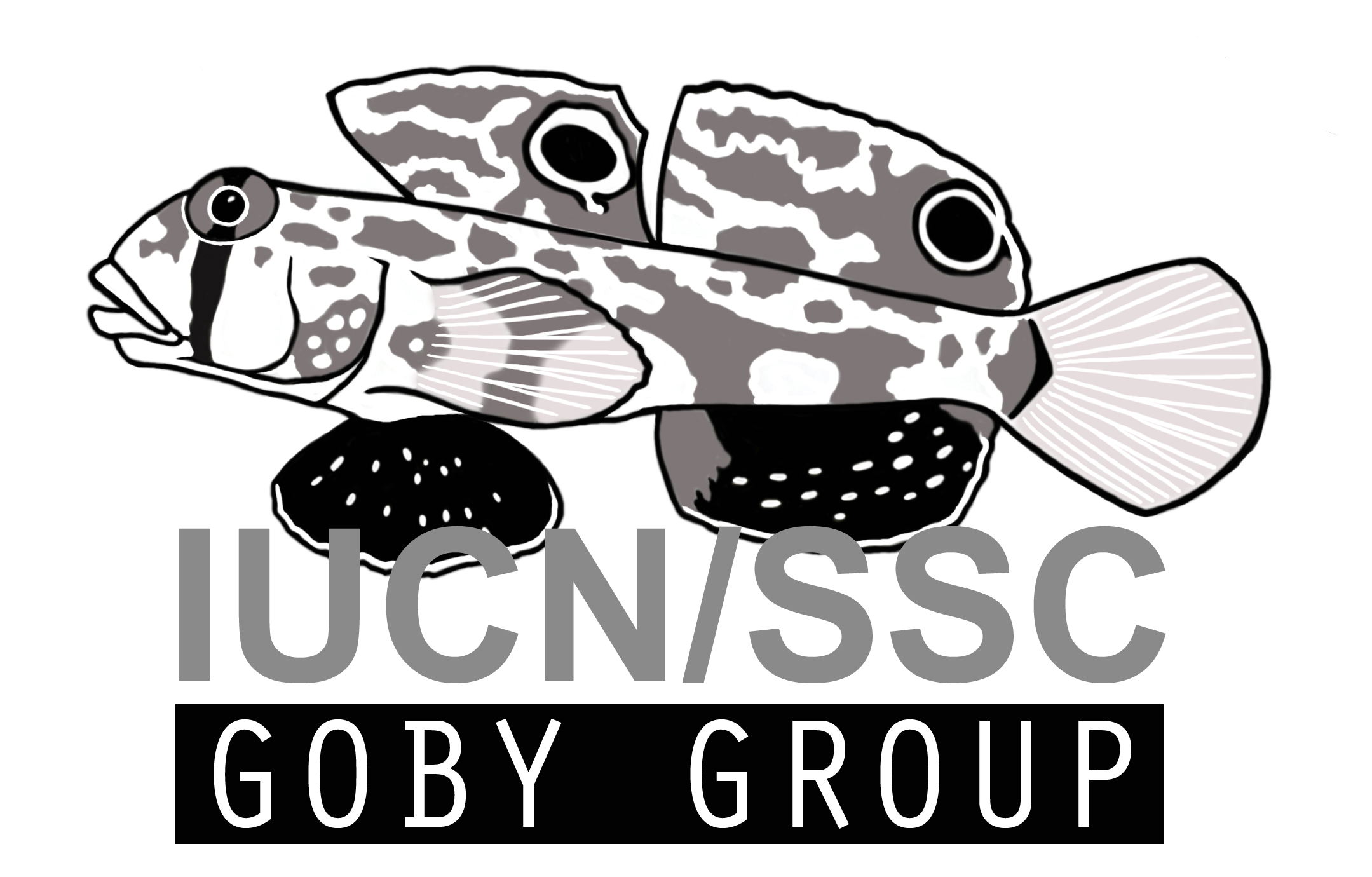This grayscale image depicts a primitive, slightly stylized drawing of a goby fish, rendered with black, white, and gray hues, including black dots and white splotches. The fish is shown in a side profile, highlighting its elongated body, five fins—two on top, two on the bottom, and one on the tail—and distinctive large white lips, with its gills detailed in black and gray. Below the fish illustration, the text "IUCN/SSC" appears in gray, followed by "Goby Group" in white on a black background. This image, potentially representing a company logo or branding element, is set against a white background and does not include any actual objects.